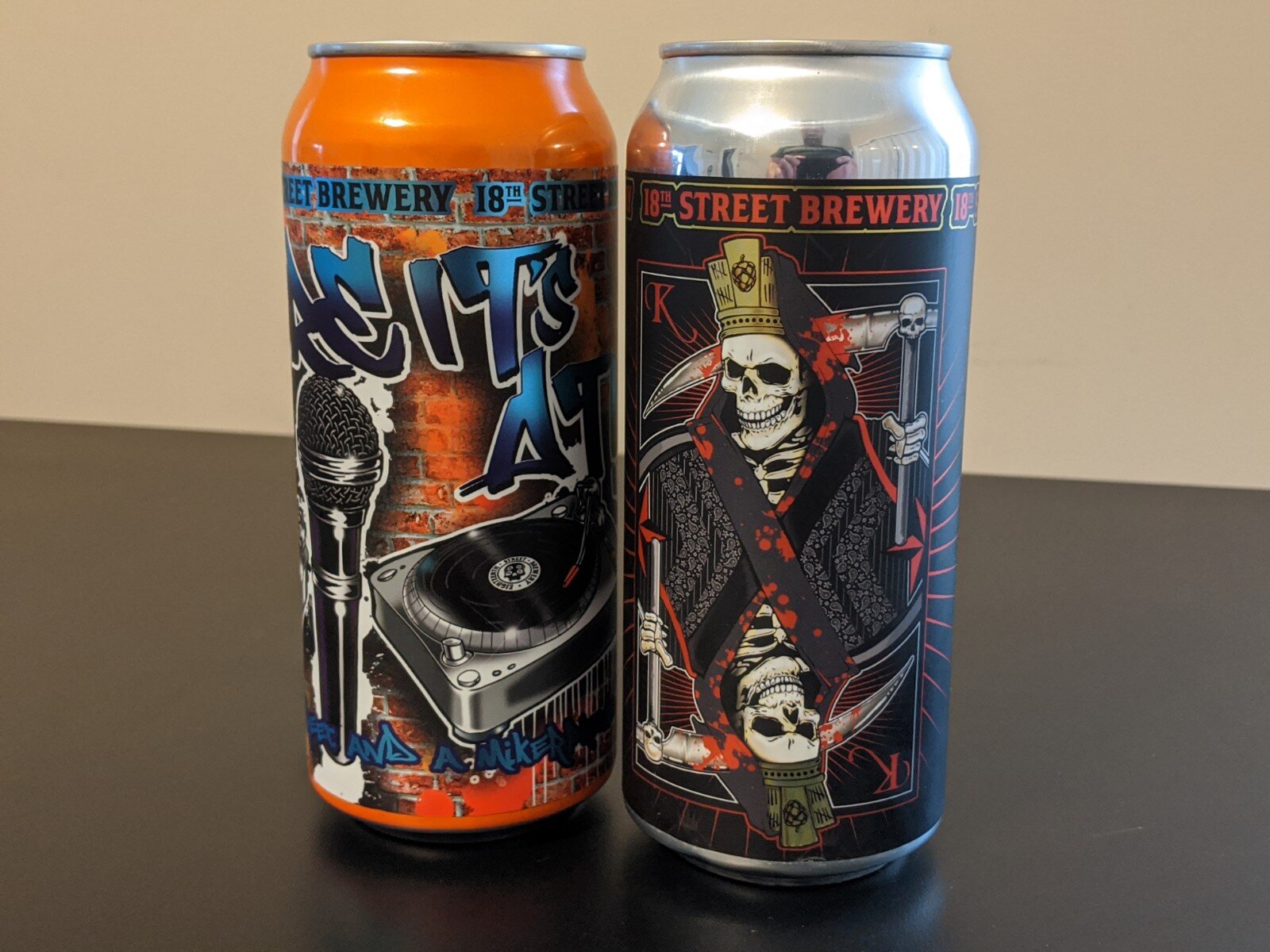The photograph shows two distinctively designed cans of alcoholic beverages from 18th Street Brewery, set on a dark table with a white background. The left can is predominantly orange and features a heavily stylized design with a large, graffiti-style font near the top, though the exact wording is unidentified. Below the text, the can showcases artwork of a microphone and a record, adding a dynamic, almost animated visual flair. The right can, in stark contrast, is silver and black, showcasing a skeletal Grim Reaper holding a scythe, reminiscent of a playing card with its mirrored composition and the inclusion of the letter 'K' at the top corners. Both cans draw attention with their bold, unique art styles, standing out sharply against the neutral backdrop.